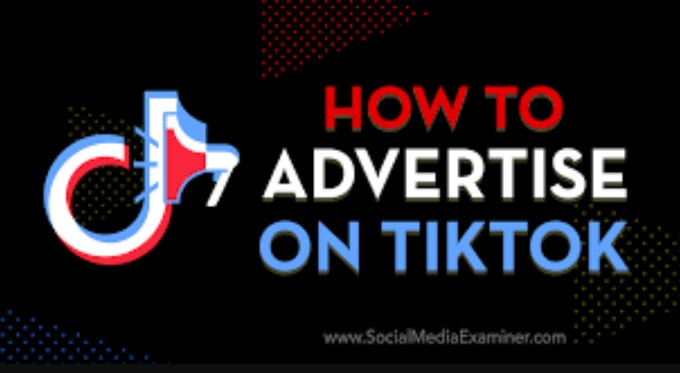This is a screenshot of a marketing banner from www.socialmediaexaminer.com. The banner exudes a distinctly patriotic theme with its dark black background complemented by striking red, white, and blue textures, suggesting it is potentially oriented towards an American audience. 

The bold headline reads "How to Advertise on TikTok" and is segmented into three lines, each with a different color scheme and font style. The first line, "HOW TO," features the TikTok logo and is capitalized and bold in red font. The second line, "ADVERTISE," is similarly capitalized and bold, but in white font. The third line, "ON TIKTOK," is capitalized, bold, and rendered in blue font. Additionally, the TikTok logo is presented in red, white, and blue, reinforcing the thematic colors.

This banner, likely intended for display on Social Media Examiner's website, serves to inform users about strategies for advertising on TikTok. It aims to attract individuals interested in learning how to effectively promote advertisements on their TikTok accounts. It targets potential users who want to recruit others and display compelling advertisements on the popular social media platform.